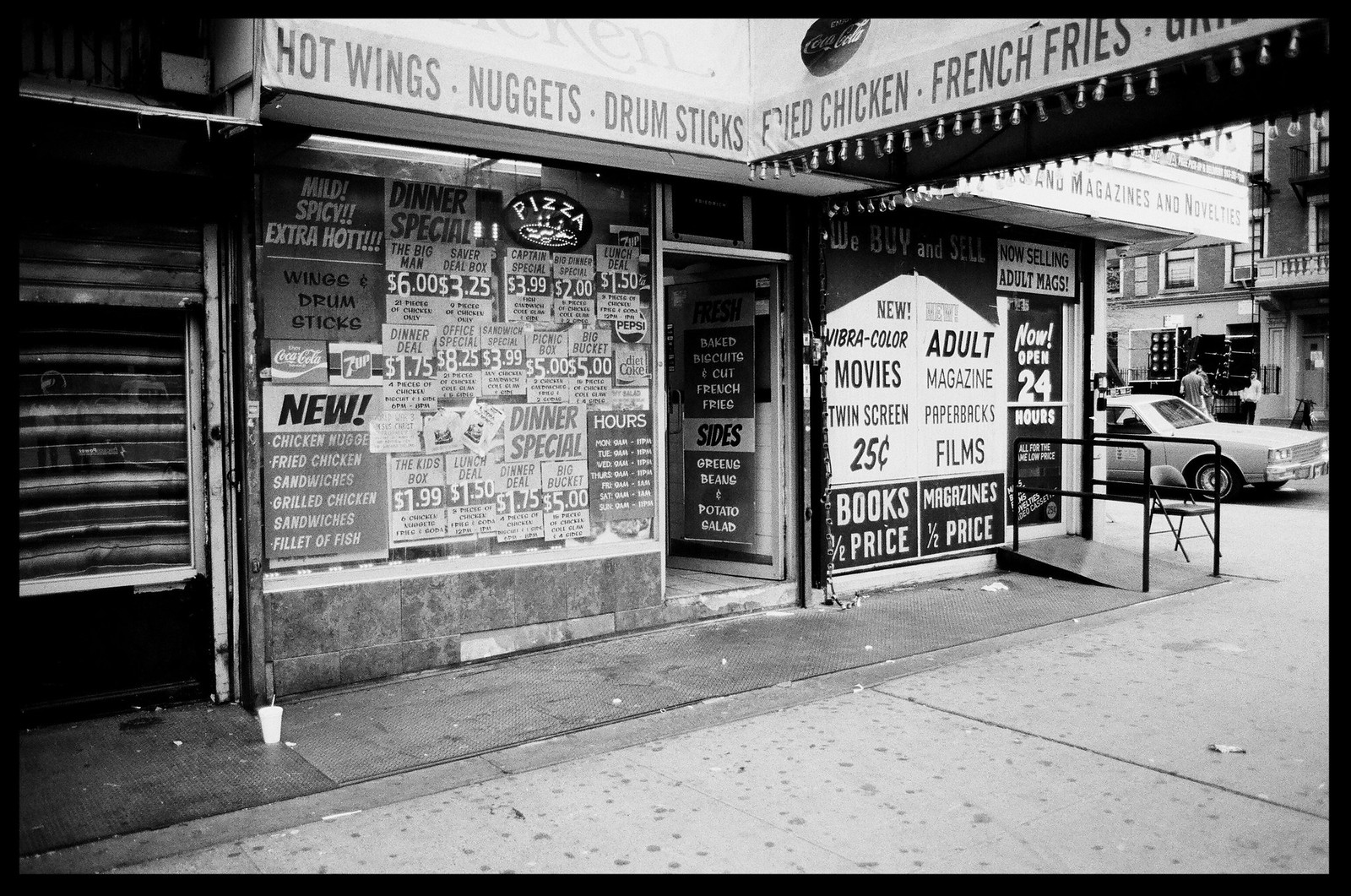This detailed black-and-white photograph, framed by a thin black border, captures a bustling corner street scene, which appears to be set in an urban environment, possibly New York City. The foreground shows a concrete sidewalk forming a triangle on the left, leading to the edge of another sidewalk on the right. Dominating the left side of the image is a storefront with an awning extending over the sidewalk, adorned with small lights reminiscent of Christmas decorations. This store, a fast-food joint, showcases a large glass window plastered with flyers and advertisements for various items, including pizza, hot wings, nuggets, drumsticks, fried chicken, french fries, a grilled chicken sandwich, and a fillet of fish sandwich. A prominent oval-shaped neon pizza sign is among the visible promotions.

Adjacent to this eatery, the right-hand section of the photograph features an adult store, identifiable by its covered windows and explicit signage promoting items such as new ultra-color movies, twin-screen films, adult magazines, paperbacks, and half-priced books. The entrance to this store is accessible via a ramp, flanked by metal bars, accommodating handicapped access. A small folding chair is noted on the sidewalk next to the ramp.

In the upper right quadrant of the image, a vintage car, likely from the 1960s or 1970s and possibly a Chevrolet, is parked on the street. Further in the distance, a pedestrian is seen peering into a store window, with an apartment building rising above. The image conveys a lively, diverse urban corner, combining elements of daily life and commerce.